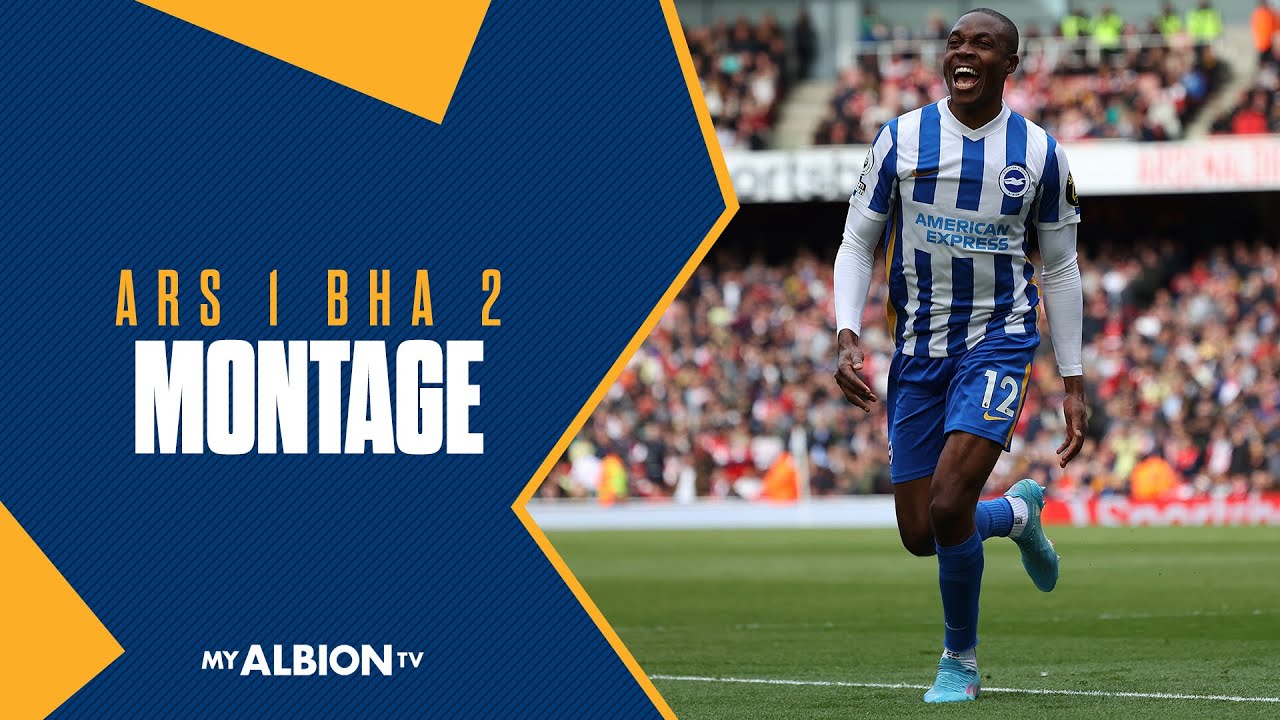The image features a joyful soccer player positioned on the right side. He is captured mid-movement, either running or walking, with a broad smile on his face. His athletic uniform is detailed with a blue and white striped jersey, white sleeves, blue shorts marked with a white number 12 and a yellow Nike symbol below, blue socks, and green shoes. The text "American Express" is emblazoned across the front of his shirt. He stands on a green field with a blurred crowd in the background. 

On the left side of the image, there is a vibrant mix of blue and orange shapes, including a zigzag outlined in orange, an orange triangle at the top, and another at the bottom left. The letters "A-R-S I B-H-A 2" are inscribed in yellow, with "Montage" written below in white, and "My Albion TV" at the bottom.